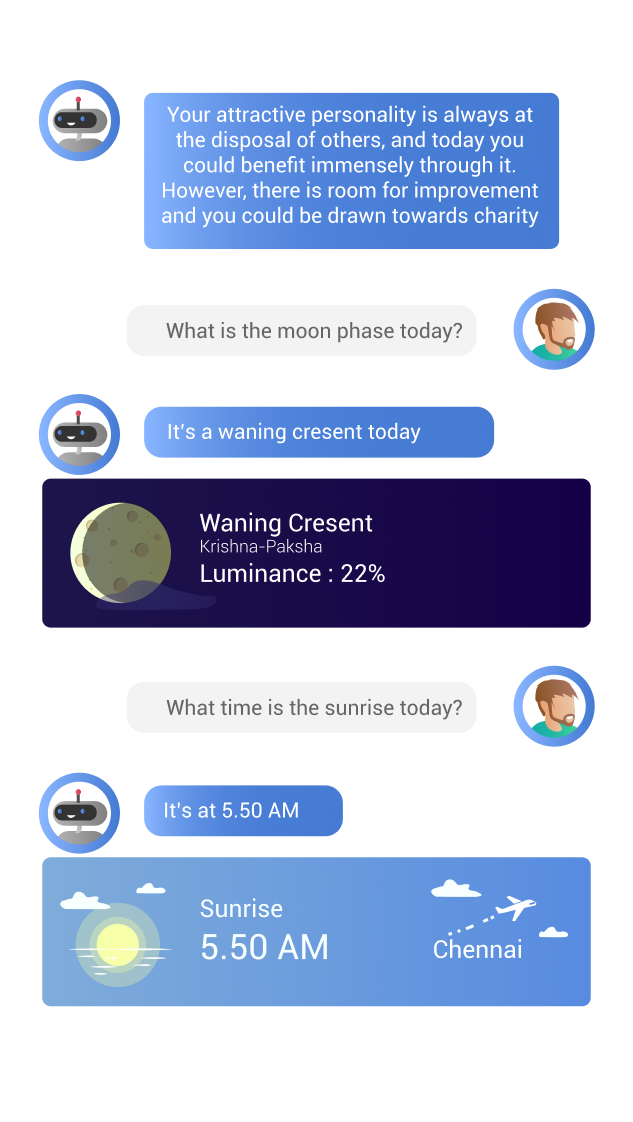Screenshot of an AI Chat Conversation:

This image captures a screenshot of a chat conversation between a user and an AI, visually represented by distinct avatars and text bubbles. 

On the left side, the AI's messages are encased in blue boxes, accompanied by an avatar of a gray robot with a rectangular head, blue eyes, a white mouth, and a red circular antenna. The first message from the AI reads: "Your attractive personality is always at the disposal of others, and today you could benefit immensely through it. However, there is room for improvement, and you could be drawn towards charity."

The user's messages appear on the right side, aligned with an avatar depicting a Caucasian man with a beard, brown hair, and wearing a green shirt. The next message shows the user's question: "What is the moon phase today?" The AI responds with: "It is a waning crescent today," followed by a visual aid—a dark blue or purple rectangular box displaying a yellow moon with only a crescent segment illuminated, indicating the "waning crescent" phase with the additional detail "Krishna Pashka, luminance 22%."

The user then inquires about the sunrise time: "What time is the sunrise today?" The AI provides the response: "It's 5:50 a.m." This is supplemented by another visual—a blue rectangular box featuring a yellow sun on the bottom left corner, white clouds, and a white airplane icon labeled "Chennai." The text next to the sun confirms "Sunrise 5:50 a.m."

Overall, this detailed screenshot showcases the interaction between a human user and a visually engaging AI, complete with helpful, contextually relevant imagery.